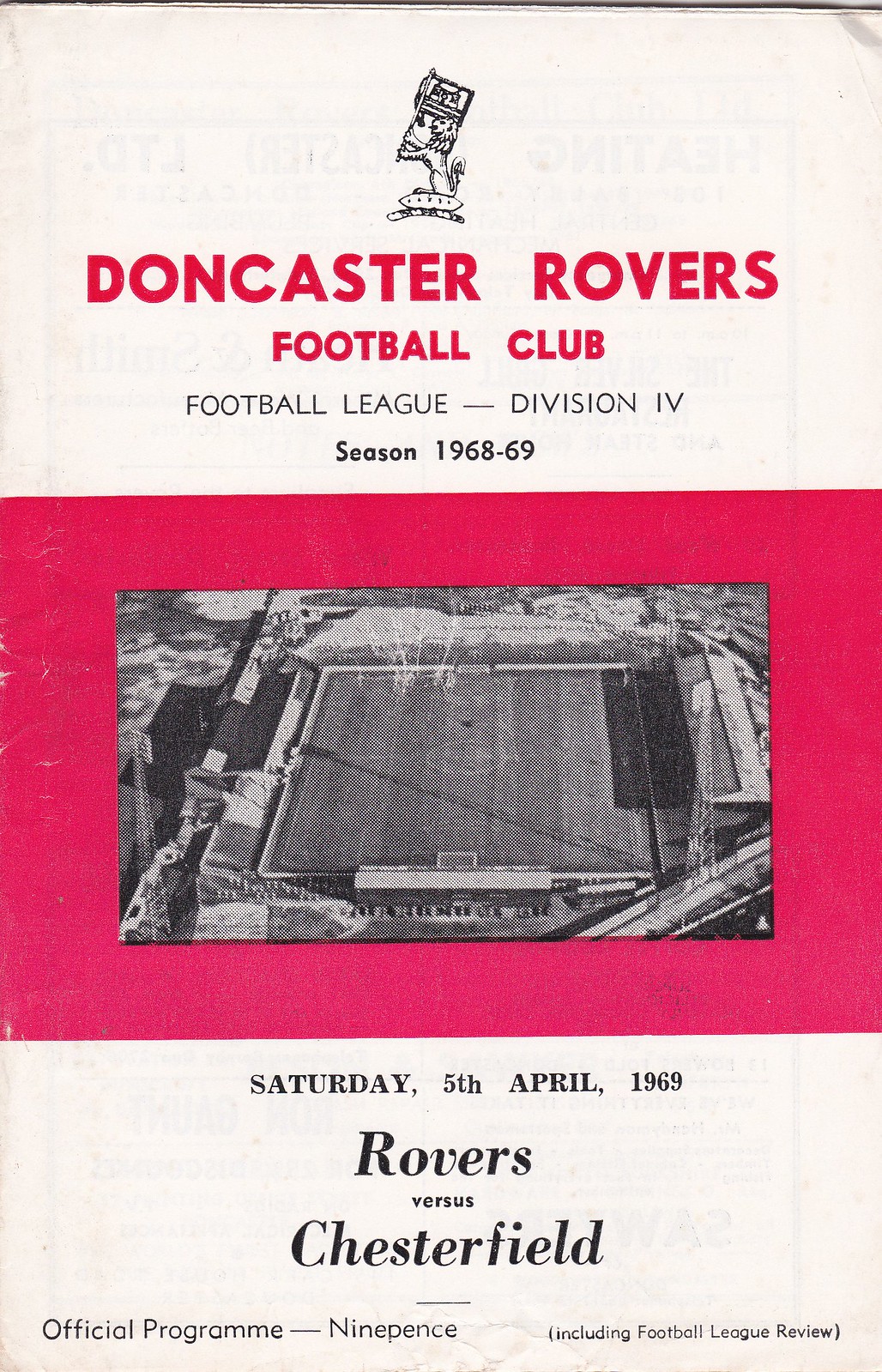This is the cover of an official program for a Doncaster Rovers football game held on Saturday, April 5th, 1969, against Chesterfield. The program is part of the 1968-69 Football League Division IV season. The cover is divided into three sections: the top third is white, featuring a logo of an animal holding a flag facing left, followed by text in red that reads "Doncaster Rovers Football Club," and in black that reads "Football League, Division IV, Season 1968-69." The central portion is dominated by a red rectangular border containing a black and white aerial photograph of the soccer stadium, with bleachers visible on both sides. The bottom third returns to a white background, displaying the event details in black font: "Saturday, 5th of April, 1969, Rovers vs. Chesterfield. Official Program, 9 pence, including Football League Review." The design predominantly features reddish, beige, and black and white colors, with the title name "Doncaster Rovers" highlighted in red at the top.